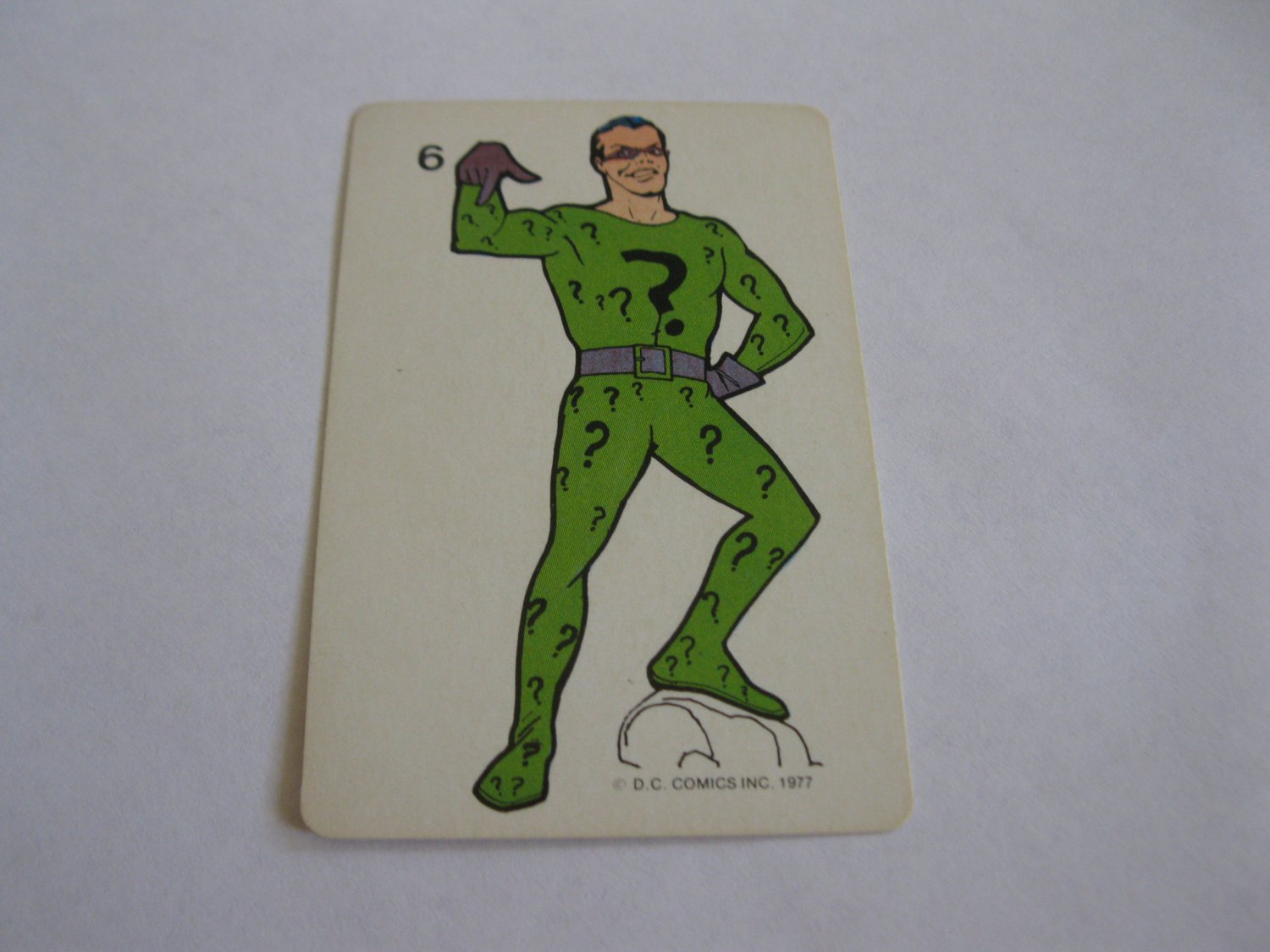The image depicts a vintage trading card placed on a flat white surface. The card, which has yellowed with age, measures as a rectangle with rounded corners and likely dates back to 1977. Centered on the card is an illustration of the Riddler, a character from DC Comics. The Riddler is wearing a green one-piece suit adorned with numerous black question marks. He sports a gray belt with a metal-looking buckle, purple gloves, and a distinctive purple eye mask. On his feet, his left foot is positioned on a rock. Notably, he has blue hair and a cheerful expression. The card's background is white, contrasting with the lighter white surface it's placed on. The card's top left corner features the number 6, and the bottom edge bears the text "© DC Comics Inc. 1977," indicating its era and origin.